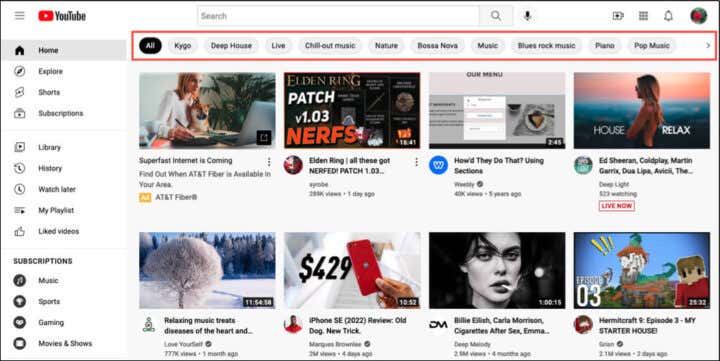The image is a detailed screenshot of a YouTube interface. In the upper left corner, the recognizable YouTube logo is displayed next to the hamburger menu icon. Adjacent to this is the search field and microphone option, while the upper right corner features various icons including the user profile, notification bell, grid view selection, and another unidentified icon.

Directly beneath this navigation bar, there is a horizontal menu highlighted by a red rectangle stretching from left to right. This menu includes categorized options such as: Hall, Kygo, DeepHouse, Live, Chillip Music, Nature, Bossa Nova Music, Blues Rock Music, Piano, and Pop Music.

Following this, the main section of the screenshot displays eight video thumbnails arranged in a 4x2 grid. Each thumbnail is accompanied by descriptive text. The titles from left to right and top to bottom include: "Superfast Internet is Coming," "Elden Ring," "How'd They Do That," "Ed Sheeran, Coldplay, Martin." On the next row: "Relaxing Music Treats," "iPhone SE," "Billie Eilish," "Carla Morrison," "Cigarettes After Sex," "Emma Something," and "Hermitcraft, Episode 3: My Starter House."

On the far left, there is a vertical menu listing options: Home, Explore, Shorts, Subscriptions, followed by a space, then Library, History, Watch Later, My Playlist, Liked Videos, and another space. Below these options, a header labeled Subscriptions appears, with further selections including Music, Sports, Gaming, and Music and Shows.

The entire screenshot is bordered by a thin black line, adding a framed finish to the captured YouTube interface.